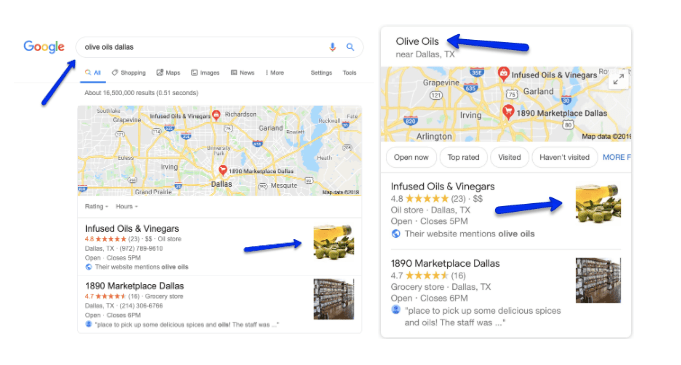The image consists of two side-by-side screenshots, both from Google Search, detailed with added blue arrows indicating specific areas within each screenshot:

1. **Left Screenshot:**
   - **Header:** The well-recognized Google logo is located at the top left corner, with "Google" displayed in its traditional blue, red, yellow, and green colors.
   - **Search Query:** The search bar at the top of the screen shows the query "Olive Oils, Dallas," highlighted by a blue arrow pointing upwards toward the search box.
   - **Map Section:** Directly beneath the search bar is a map displaying several pins, each representing a different olive oil business in Dallas.
   - **Business Listings:** Below the map, a list of businesses corresponding to the pins is visible. The first listed business is "Infused Oils and Vinegars," which is emphasized by a blue arrow pointing to its thumbnail image.

2. **Right Screenshot:**
   - **Search Header:** At the top, the words "Olive Oils" are presented prominently, with a blue arrow drawing attention to this header.
   - **Location Description:** Under the search header, the text "near Dallas, Texas" is visible, indicating the geographical focus of the search.
   - **Zoomed-In Map:** A map similar to the one in the left screenshot is displayed but zoomed in for greater detail.
   - **Business Highlight:** Another blue arrow, positioned below the "Infused Oils and Vinegars" section, again points to the thumbnail image associated with this business, mirroring the emphasis seen in the left screenshot.

These screenshots collectively showcase a detailed search experience for olive oil offerings in Dallas, with particular focus on the "Infused Oils and Vinegars" business, as indicated by the blue arrows.